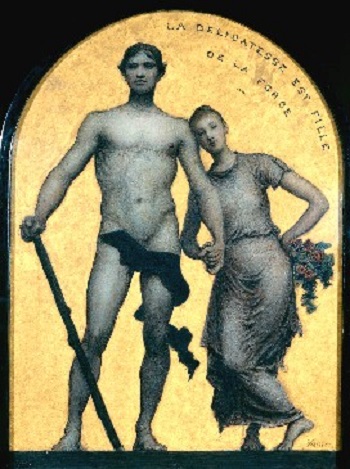The artwork is a vertical, rectangular piece, featuring a painted or drawn style with digital influences. Set against a black background, a soft gold arched rectangle dominates the composition. The arch bears a French inscription: "La délicatesse est fille de la foule." In front of this arch stand a man and a woman holding hands, with the man on the left and the woman on the right.

The man is nearly naked, wearing just a black strip of cloth around his groin and left thigh, and holds a staff diagonally to the ground in his right hand. He stands upright. The woman, leaning gently against his shoulder, wears a light-colored dress with short sleeves, which reaches her ankles. Her legs are crossed, and she holds a bouquet of flowers in her left hand, her elbow crooked and the bouquet pointed downward. The flowers include green stems with faint red roses. There are no other people or additional text in the image.